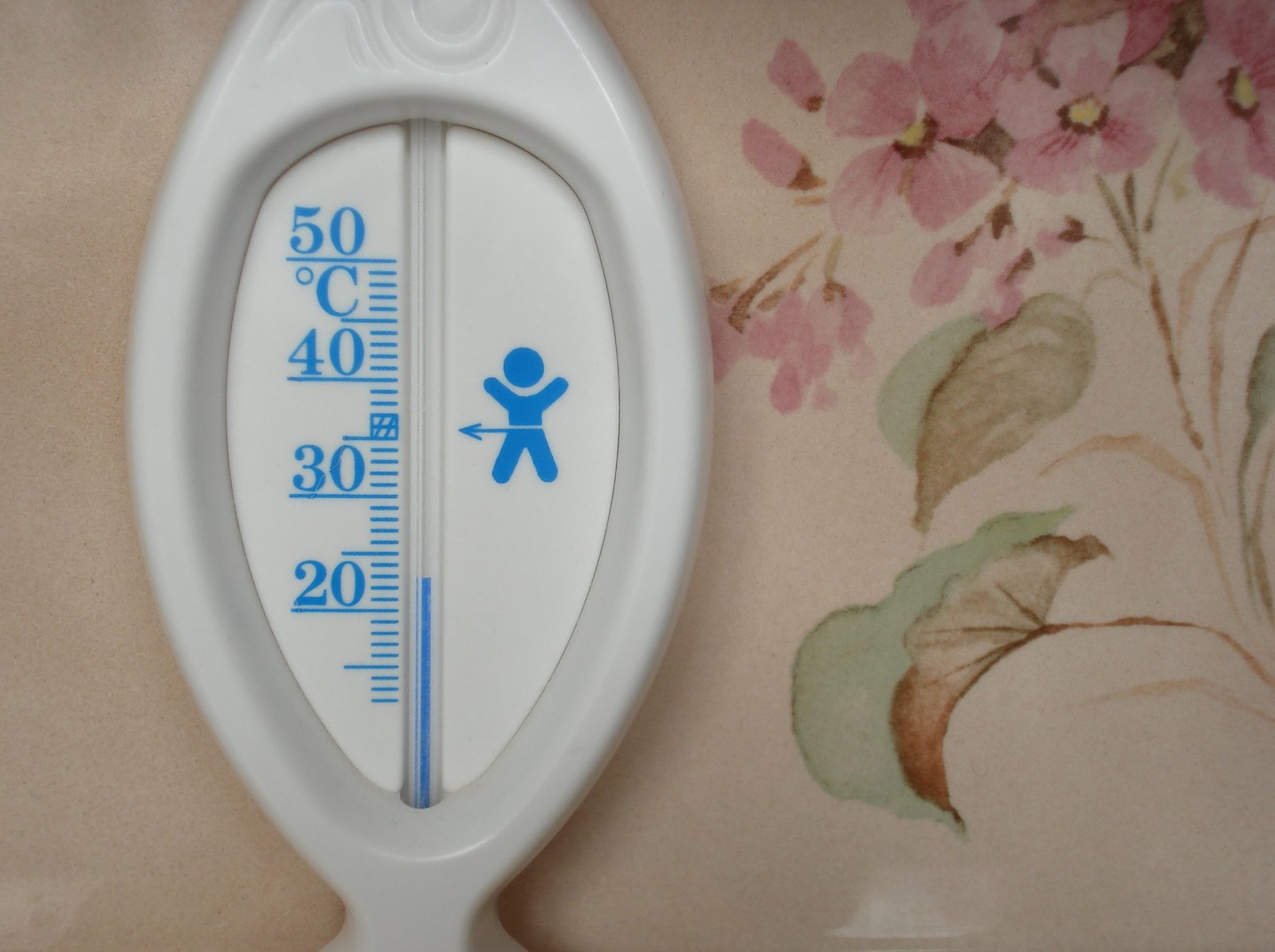In the photograph, the backdrop showcases an off-white tablecloth adorned with a simple floral pattern situated in the upper right corner. The design features three grayish flowers, each with four petals and vibrant yellow centers. The flowers are connected by green stems, along with two green leaves adding to the natural detail.

The central focus of the image is a plastic-framed thermometer, prominently displayed in an oval, white enclosure. The thermometer is calibrated in Celsius. The left side of the thermometer vertically lists temperature markers: 50, followed by a long blue line, then the letter "C" representing Celsius. Beneath "C," the scale continues with numerical increments of 40, 30, and 20, descending in blue dashes towards the bottom of the thermometer.

The core of the thermometer features a thin vial filled with blue liquid, designed to measure temperature accurately. On the right side of the thermometer’s face is a small, blue icon of a humanoid figure with arms raised, symbolizing a human form. This visual composition underscores the functional yet simplistic design of the thermometer, set against a subtly decorative background.